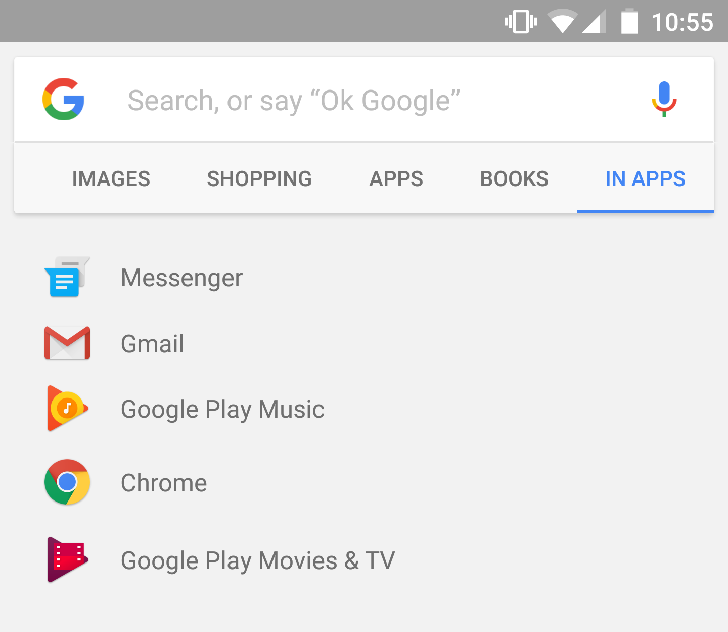In this close-up view of a smartphone screen, the top section features a grey status bar. On the right side of the bar are several icons: 

1. An unidentified icon consisting of two lines on both the left and right sides of a square, possibly representing a mobile signal.
2. The Wi-Fi signal icon, which shows a strong but not full connection.
3. The cellular signal icon, also indicating a fairly strong but not full signal.
4. A fully charged battery icon.
5. The current time displayed as 10:55.

Below the grey status bar, there's a Google search bar with a multicolored "G" logo (red, yellow, green, blue) and the text "Search or say 'OK Google.'" To the right of this text is the Google microphone icon.

Under the search bar are several navigation options: "Images," "Shopping," "Apps," "Books," and "In Apps." The "In Apps" option is selected, highlighted with a blue underline.

Further down, the screen shows an array of app icons:
1. A blue and white document icon labeled "Messenger."
2. A white envelope with red trim labeled "Gmail."
3. A red triangle with an orange circle and a musical note, representing "Google Play Music."
4. A camera lens icon with red, yellow, and green segments encircling a blue center, representing "Chrome."
5. A red triangle with a red film strip labeled "Google Play Movies & TV."

The background color beneath the grey banner transitions to a light grey or off-white shade.